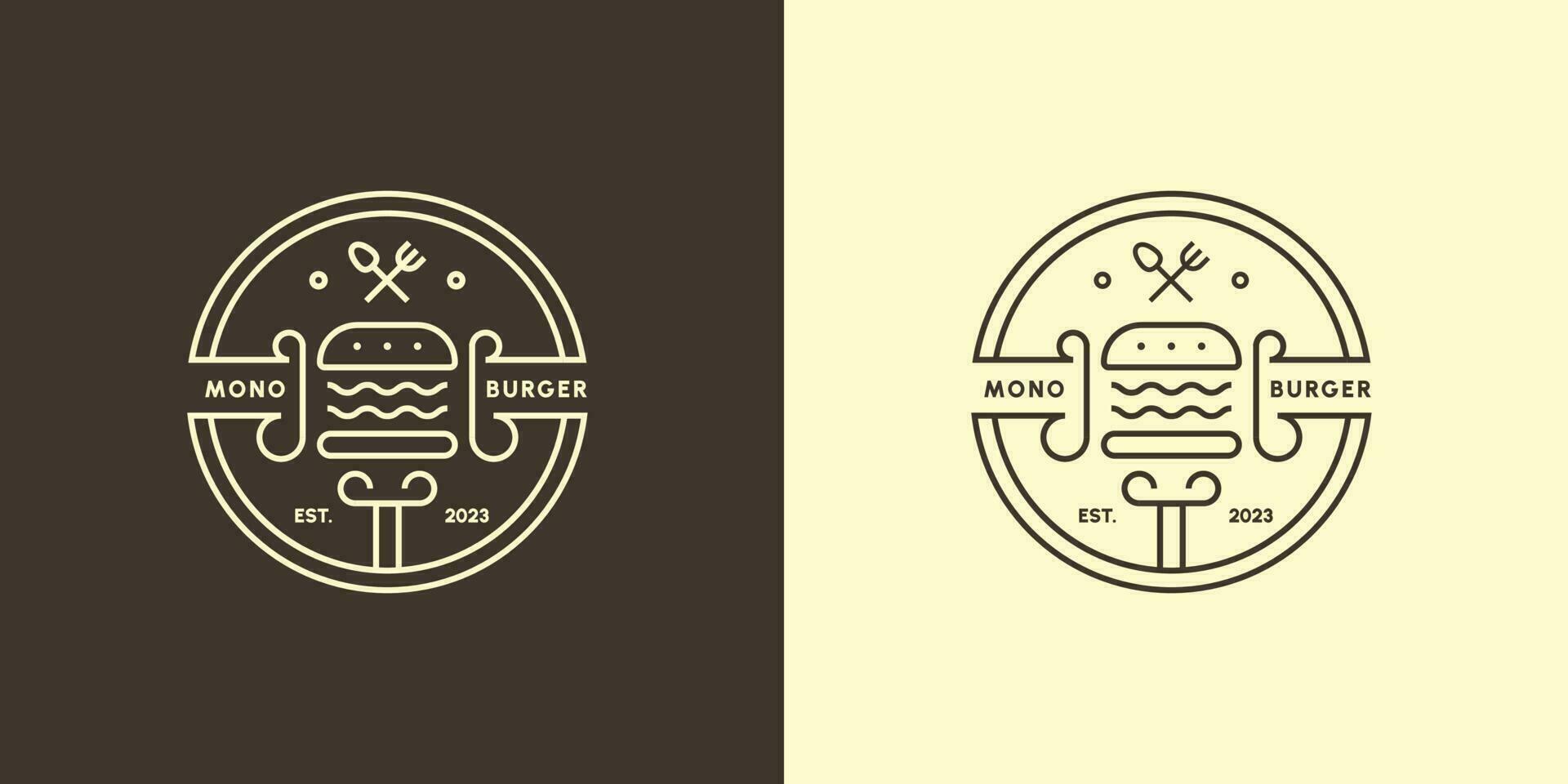The image features a business logo depicted twice side by side, with inverted color schemes. On the left, the logo is rendered in white lines on a black background, and on the right, it is shown in black lines on a cream-colored background. The logo itself is a circular design with a stylized hamburger in the center, topped by crossed spoon and fork symbols. To the left of the hamburger, it reads "Mono," and to the right, it says "Burger." Below the burger, there is a scroll-like element with the text "EST" on the left and "2023" on the right, signifying the establishment year. Additionally, two small dots flank the crossed spoon and fork at the top of the circle. The overall presentation is clean and modern, using contrasting colors to create a visually appealing and memorable brand image.